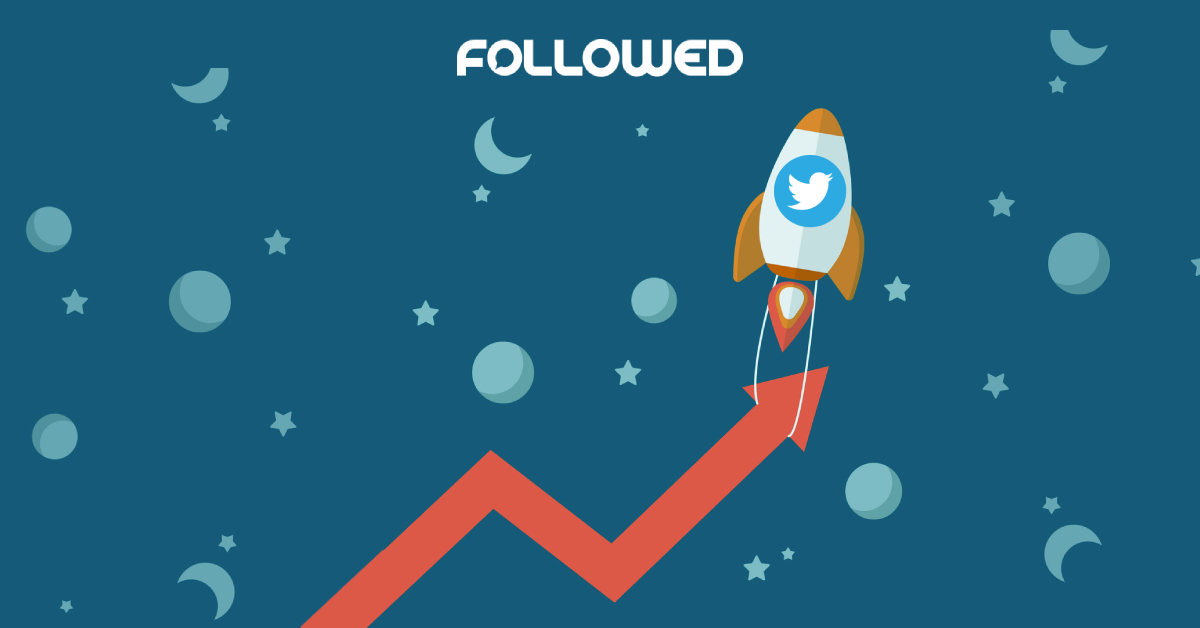This horizontal color illustration features a vibrant, dynamic scene set against a gradient blue background. The background is predominantly a dark, dull blue but transitions to a slightly greener shade at the bottom right corner. Dominating the top portion of the image, the word "FOLLOWED" is prominently displayed in large, white bubble text.

Near the center of the illustration, a stylized rocket ship emoji captures attention. This rocket is predominantly white and gray, adorned with orangish-yellow wings and showcasing the iconic Twitter logo at its center. Fiery exhaust shoots from its rear, emphasizing motion and energy.

Emerging from the bottom left quadrant, a red zigzag arrow snakes upward, dips downward, and ascends again, leading the eye toward the rocket. A thin white cord wraps around and behind the top part of the arrow, seemingly tethering the rocket to its path.

The background is speckled with celestial elements, including small stars and round planets or moons. These planets display a dual-tone color scheme, with light blue on one half and a darker blue on the other, adding depth and a sense of cosmic wonder to the scene.